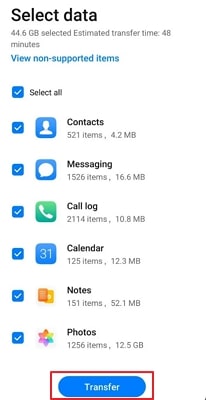The image depicts a transfer section on a smartphone screen with a clean, white background. At the top, the bold text "Select Data" stands out in black. Beneath this header, the display indicates "44.6 GB selected" with an estimated transfer time of 48 minutes. There is also an option to "View non-supported items." Below this, a checkbox labeled "Select All" is marked, signifying that all transferrable items are selected.

The screen lists specific categories of data to be transferred, starting with:
1. Contacts: 521 items, totaling 4.2 MB.
2. Messaging: 1,526 items, totaling 16.6 MB.
3. Call Log: 2,114 items, totaling 10.8 MB.
4. Calendar: 125 items, totaling 12.3 MB.
5. Notes: 151 items, totaling 52.1 MB.
6. Photos: 1,256 items, totaling 12.5 GB.

At the bottom of the screen, the "Transfer" button is highlighted in blue and outlined with a red box, emphasizing its importance in the image.